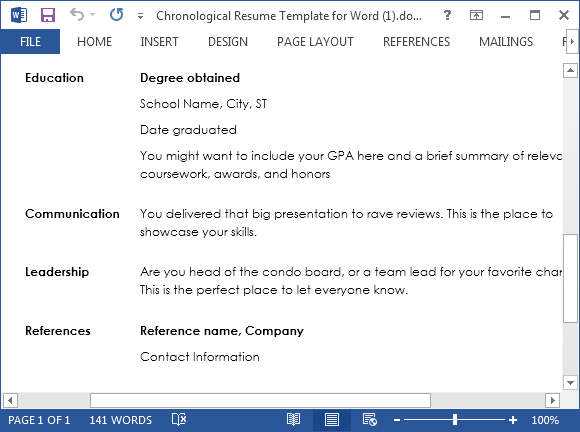**Detailed Caption:**

This image is a screenshot taken from a computer displaying a "Chronological Resume Template for Word". The template is primarily rectangular with a white background and black text. At the top, small text reads "Chronological Resume Template for Word #1," followed by "do..." and a question mark, accompanied by various symbols situated in the upper left and right corners. 

A large blue rectangle highlights the word "File" in the taskbar, indicating that the user has clicked this option. Below, the template is organized into different categories: 

1. **Education**: This section prompts the user to enter details such as the degree obtained, the school name, city, state, and the graduation date. It suggests including the GPA for emphasis.

2. **Communication**: Here, users are encouraged to detail notable achievements, such as delivering a significant presentation, with an emphasis on showcasing skills.

3. **Leadership**: This section asks the user to divulge any leadership roles, such as being the head of a condo board or a team lead, making it the perfect place to highlight leadership experience.

4. **References**: Users are prompted to provide the names of references along with their company and contact information.

This resume template acts as a guided framework for users to fill in their personal and professional information, aiding them in creating a detailed and organized resume.